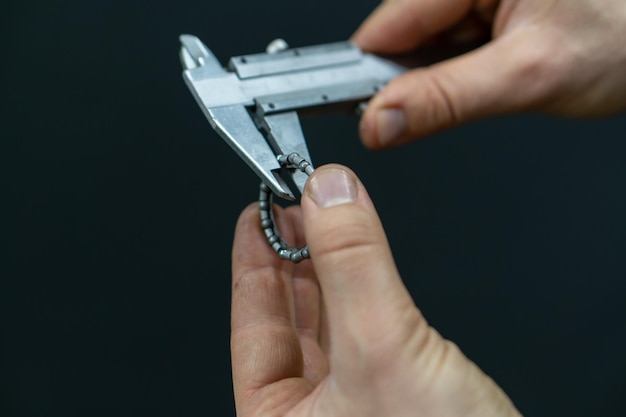In the image, a man is meticulously measuring a small, bumpy ring with a pair of calipers. The ring, adorned with spherical beads separated by about the length of two beads, is held securely in his left hand while the calipers, manipulated by his right hand, grip one bead section. Despite the focus on his left hand, which reveals a slightly dirty index finger possibly marked with tread or wrinkles, his right hand appears blurred in motion. The metal caliper, which resembles a small silver ruler with a hammerhead, is used for precision measurement, though it is difficult to discern the exact dimension due to the blurred focus on the calipers. The background is a stark, solid black, emphasizing the vivid, focused details of the measuring process while the man’s thumb and index finger clasp the caliper's end.